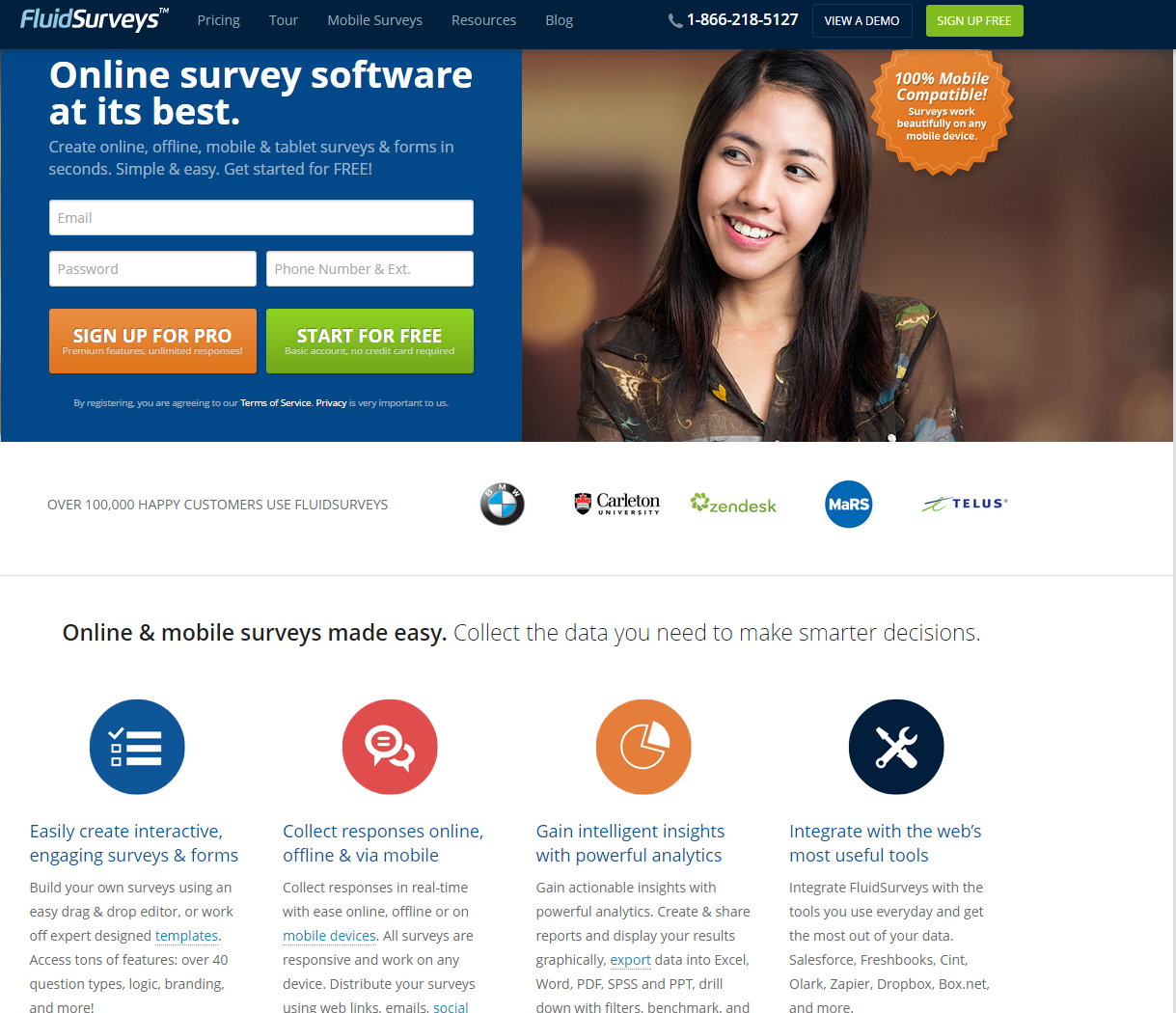The image features a promotional design for Fluid Surveys, emphasizing its ease of use and robust feature set. The central section highlights the trust and satisfaction of over 100,000 happy customers, with notable clients including BMW, Call to Action University, Zendesk, Mars, and TELUS. This section includes testimonials and is overlaid on a white background with a thin gray line at the bottom, dividing the segments clearly.

Below the main testimonial section, the caption reads: "Mobile, online mobile surveys made easy. Collect the data you need to make smarter decisions." Following this, there are visually distinct circular icons providing a breakdown of Fluid Surveys' features:

1. **Blue Circle**: "Easily create, engage, and service your forms."
2. **Red Circle**: "Collect responses online or via mobile." Within this icon, a text box stands out in white.
3. **Orange Circle**: Features a white pie chart, expanding on the idea: "Gain intelligent insights with powerful analytics."
4. **Navy Blue Circle**: Exhibits a wrench and screwdriver in white, with the text: "Integrate with the web's most useful tools."

Bordering the top of the image is a blue strip reading "Fluid Surveys" in white, accompanied by navigation options in light blue: "Pricing," "Tool," "Mobile Surveys," and "Resources." 

A contact number is prominently displayed: "1-866-218-5127," which is in white against the blue background. Adjacent to this is a green box with the prompt "View a demo," while another prompt "Sign Up Here" follows. Additional promotional text includes: "Online survey software at its best," and the tagline: "Create online or mobile and tablet surveys and forms in seconds. Simple and easy. Get started for free." All text elements maintain a clear and accessible color scheme, ensuring that the key benefits and calls to action are immediately visible and understandable.